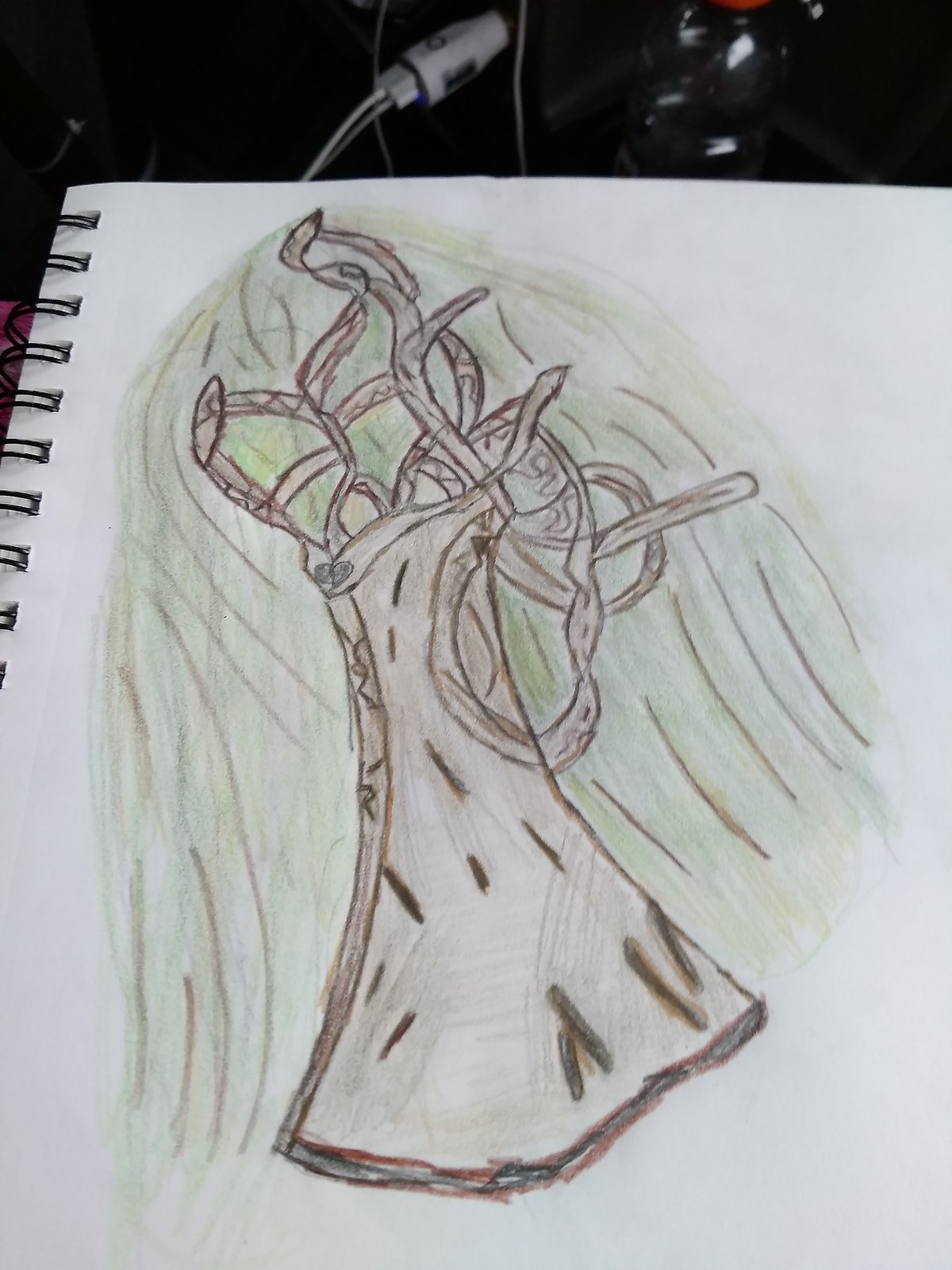The image features a detailed drawing on a white sheet of paper from a spiral-bound notebook. The focal point of the artwork is a tree trunk with branches contorted in various directions. The tree is primarily colored in light brown, with the background subtly shaded in light green, adding texture and depth. Intriguingly, some of the branches possess characteristics resembling snake heads and patterns, suggesting a 'snake tree' with branches that could be interpreted as serpents. There are also grayish shading lines enhancing the drawing's depth. Behind the notebook, the background reveals some plugged-in cords or a car charger, and a darker room ambiance. The image gives off a sense of nature intertwined with imaginative, almost fantastical elements, like tentacle-like straps or snake-like branches, contributing to an overall eerie or mystical feel.